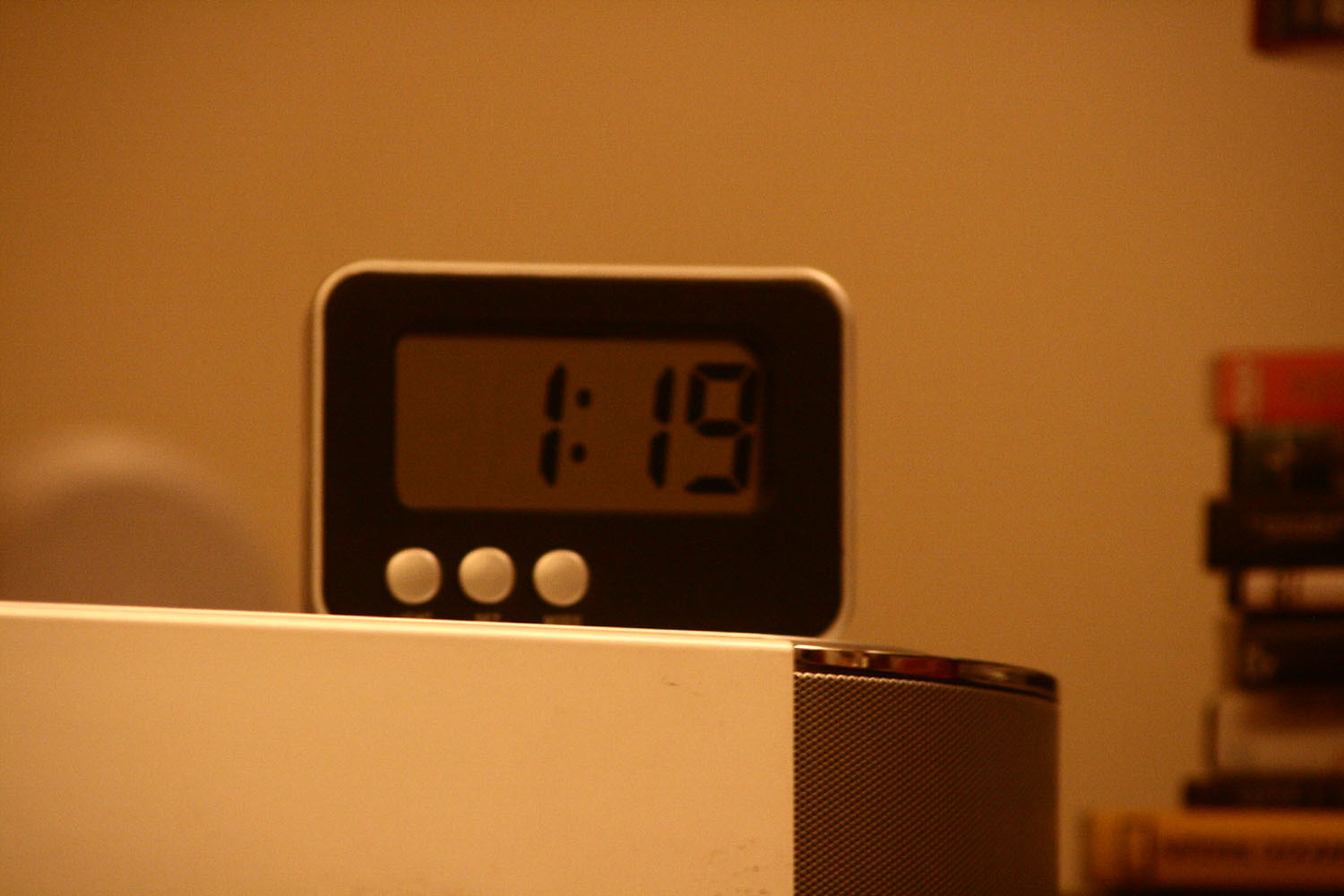The image depicts a dimly lit room with a distinct orange or yellowish tint, suggesting it might be someone's home. At the center of the foreground, there's a small digital alarm clock displaying the time "1:19." The clock features a black face with black digital numbers and a border that transitions from black to white at the very edges. It has three white buttons on the bottom left, though the labels are difficult to decipher. The clock is perched on a white, rounded object that resembles a speaker, with a silver mesh front designed for sound output. In the background, on the right side of the image, there is a stack of approximately seven to ten differently-sized and colored books. The walls of the room appear to be white or off-white with an orange or brownish tint, enhancing the room's cozy, somewhat nostalgic ambiance.